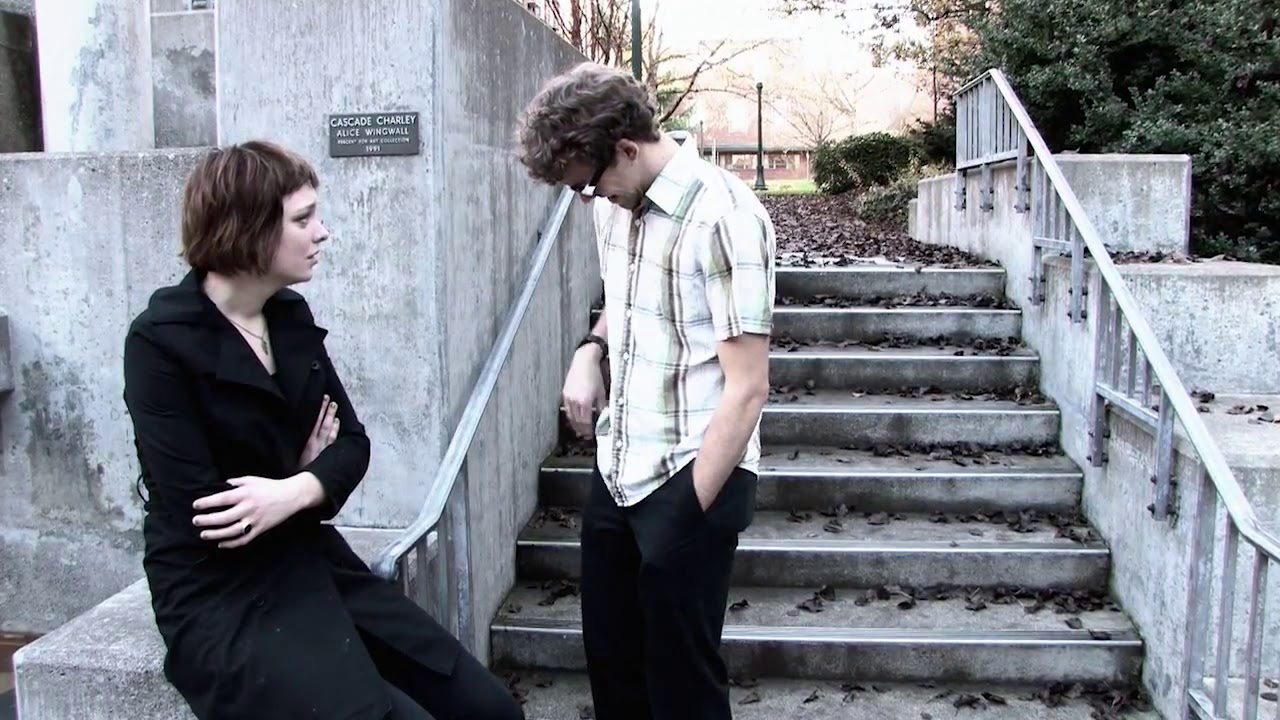In the image, an outdoor scene unfolds at the bottom of a concrete staircase that is scattered with fallen leaves, suggesting it is autumn. The sky in the background hints at the setting sun, creating a serene yet slightly chilly atmosphere. On the left side of the stairway, a woman is seated on the stone step near a railing. She has short brown hair and is dressed entirely in black, possibly a peacoat and pants. Her arms are folded across her chest as she engages in conversation with a young man standing to her right. The man, who has wavy brown hair and wears black-framed glasses, is dressed in a white and black plaid short-sleeved button-down shirt and black pants. He wears a black watch on his right wrist and keeps his left hand in his pocket, seemingly looking downwards. Behind them, a concrete wall displays a plaque reading "Cascade Charlie Alice Wingwall," with more details that are unreadable from this angle. Surrounding the stairway are trees, with some visible lampposts in the distant background, adding to the tranquil yet somber feel of the setting.